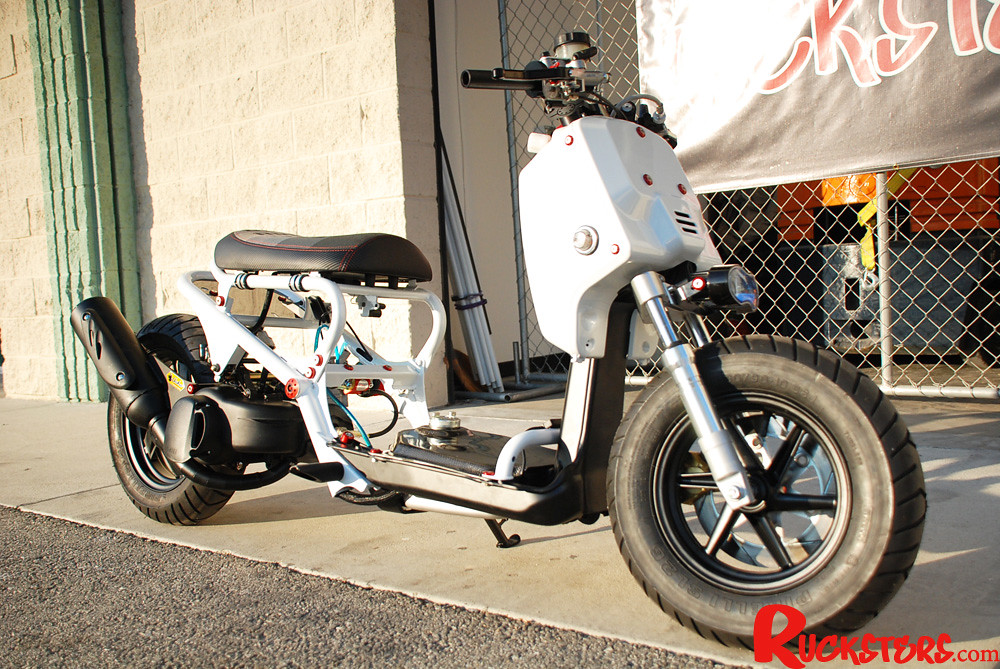This outdoor daytime photograph features a low-slung, white scooter with a black seat and black tires, parked on a sidewalk bordering a gray road. The scooter, which resembles a simplified motorcycle or moped, includes a black handlebar and an upward-tilted black muffler. It is characterized by a distinctive white frame, with the letter "C" in orange on it, and prominently features the text "Rucksters.com" in red in the lower right-hand corner of the image. The background reveals a chain-link fence with a partially visible sign containing the letters "CKS," a green pillar, some metal poles leaning against a wall, and a cinder block building to the left. The scooter, which seems to be equipped for moderate speeds and has a kickstand to prevent it from falling, is angled slightly rather than positioned straight on in the frame.